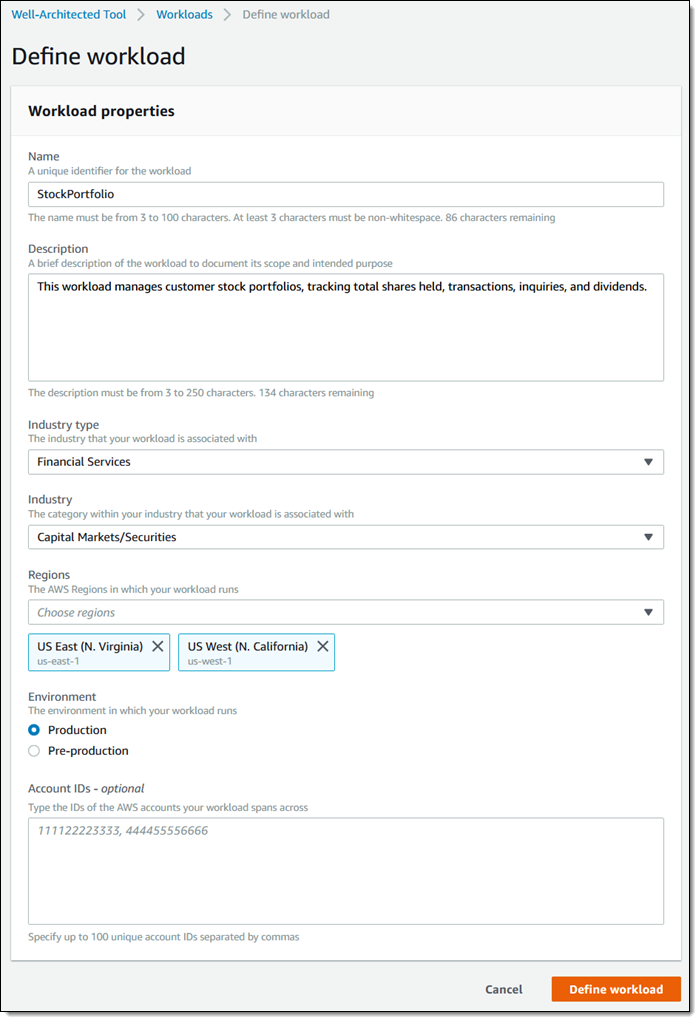The web page displayed is for defining a workload using the Well-Architected Tool. At the top, the page title reads "Define Workload," accompanied by a right-facing arrow and the phrase "Workloads." 

**Define Workload**:
1. **Workload Properties**:
   - **Name**: The input box contains the unique identifier "stockportfolio" (entered as a single word).
   - **Description**: A detailed description explains the workload's purpose: "This workload manages customer stock portfolios, tracking total shares held, transactions, inquiries, and dividends."
   
2. **Industry Type**:
   - A dropdown menu is used here, and "Financial Services" is selected.
   
3. **Industry**:
   - Another dropdown provides the selection for "Capital Markets / Securities."
   
4. **Regions**:
   - For this field, there's a prompt to choose a region with no selection made yet. However, predefined regions include:
     - US East (Northern Virginia) - us-east-1
     - US West (Northern California) - us-west-1
   - These selections appear in a light blue box with a blue border and can be closed out if not needed.

5. **Environment**:
   - Two radio buttons are available: "Production" and "Pre-production," with "Production" currently selected.
   
6. **Account IDs (Optional)**:
   - A series of account IDs is listed: 1111-2222-3333, 4444-5555-6666.

At the bottom of the page, there are two action buttons: "Cancel" and "Define Your Workload."